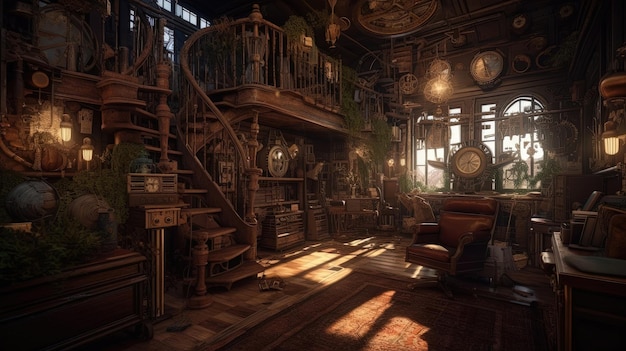The image appears to be a highly detailed, dimly lit, indoor scene that resembles an old house or possibly a computer-generated setting from a video game. The entire space is constructed from dark brown wood, creating a warm yet mysterious atmosphere. A wooden staircase with an intricate banister loops around the left-hand side, adorned with some plants that also appear sporadically on the right. In the middle of the room stands a brown leather chair. To the right, near a window that allows a stream of sunlight to pierce the otherwise dim room, sits a desk. Clocks and clock gears are scattered throughout the room, notably one on the desk and another positioned above the window. The walls and various surfaces are teeming with knickknacks and odd items, giving the impression of either a clock collector’s haven or an antique clock shop. Lanterns provide additional subdued lighting, enhancing the intricate detailing and cozy yet cluttered ambiance of the space.